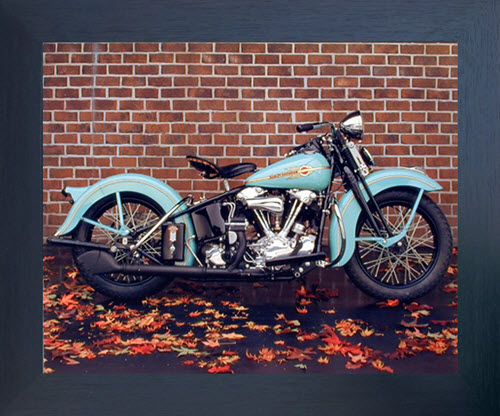In this detailed image, a robin's egg blue Harley-Davidson motorcycle with gold stripe accents stands proudly against a red brick wall backdrop. The bike features silver chrome components including the engine block, headlamps, and handlebars, while the body and pipes are painted black. The motorcycle, showcasing its black tires and black seat cushion, is surrounded by a scattering of autumn leaves in hues of red, brown, orange, yellow, and peach. The surface beneath appears to be black or dark gray, adding to the outdoor setting's autumnal feel. Framed in a black wooden frame, this portrait captures the timeless elegance and rugged appeal of the classic Harley-Davidson.